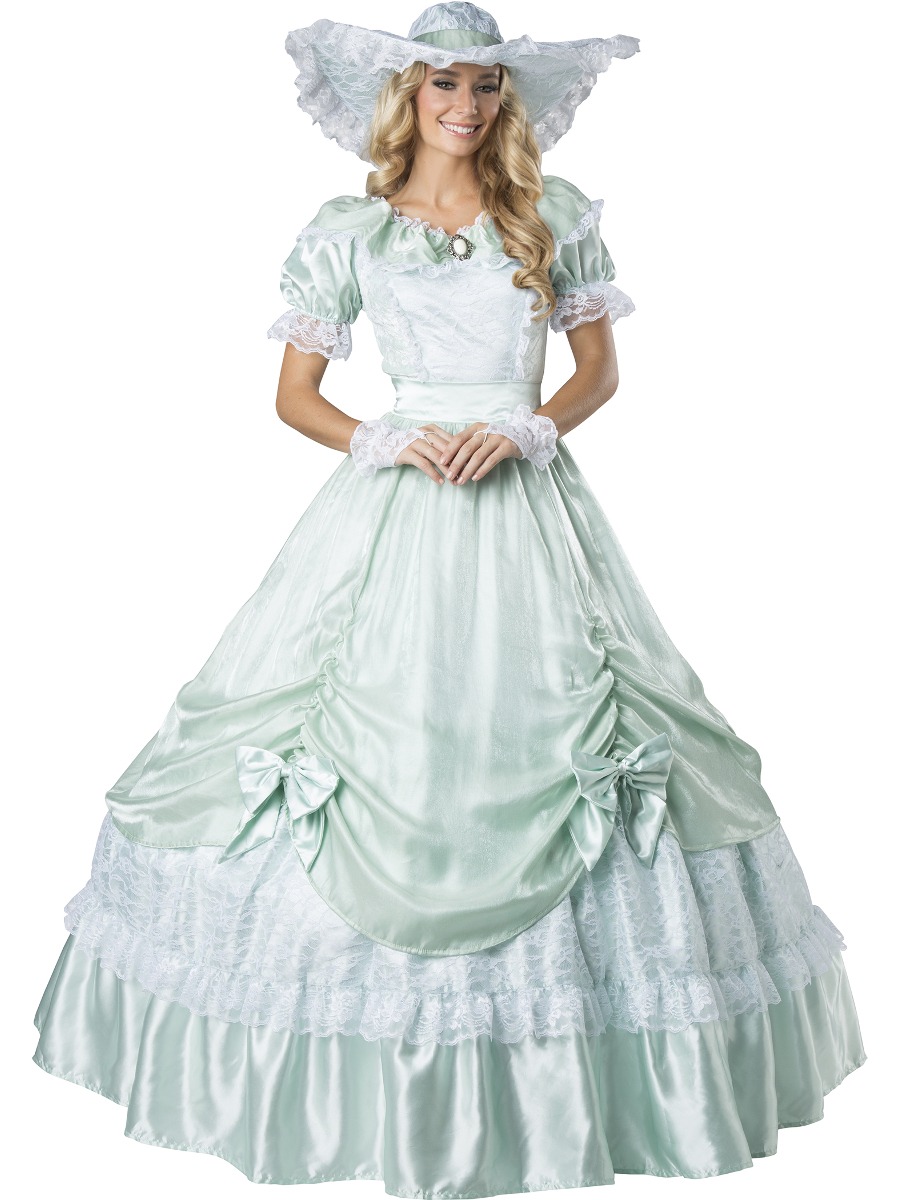This photograph features a gorgeous Caucasian woman with long, wavy, blonde hair cascading over her shoulders and down her back. She is dressed in an elegant, Victorian-inspired gown that is a very light turquoise or blue color. The gown is adorned with intricate white lace detailing and has a wide, poofy skirt that flares out from her waist, featuring a couple of bows partway up the bottom. She accessorizes with lace fingerless gloves that extend to her wrists, adding a touch of vintage charm.

Her attire is complemented by a stylish broad-brimmed hat decorated with a light blue ribbon just above the rim. The hat elegantly frames her face, which is illuminated by a bright, inviting smile. At the neckline of the dress, she wears a distinctive brooch that accentuates the dress’s sophisticated scooped neck design.

The woman's overall look is one of timeless elegance, reminiscent of a Southern Belle or a figure from the Victorian era, suggesting she is either attending a formal event or perhaps posing for a themed photoshoot. The white background focuses attention on her striking appearance and meticulously coordinated outfit.